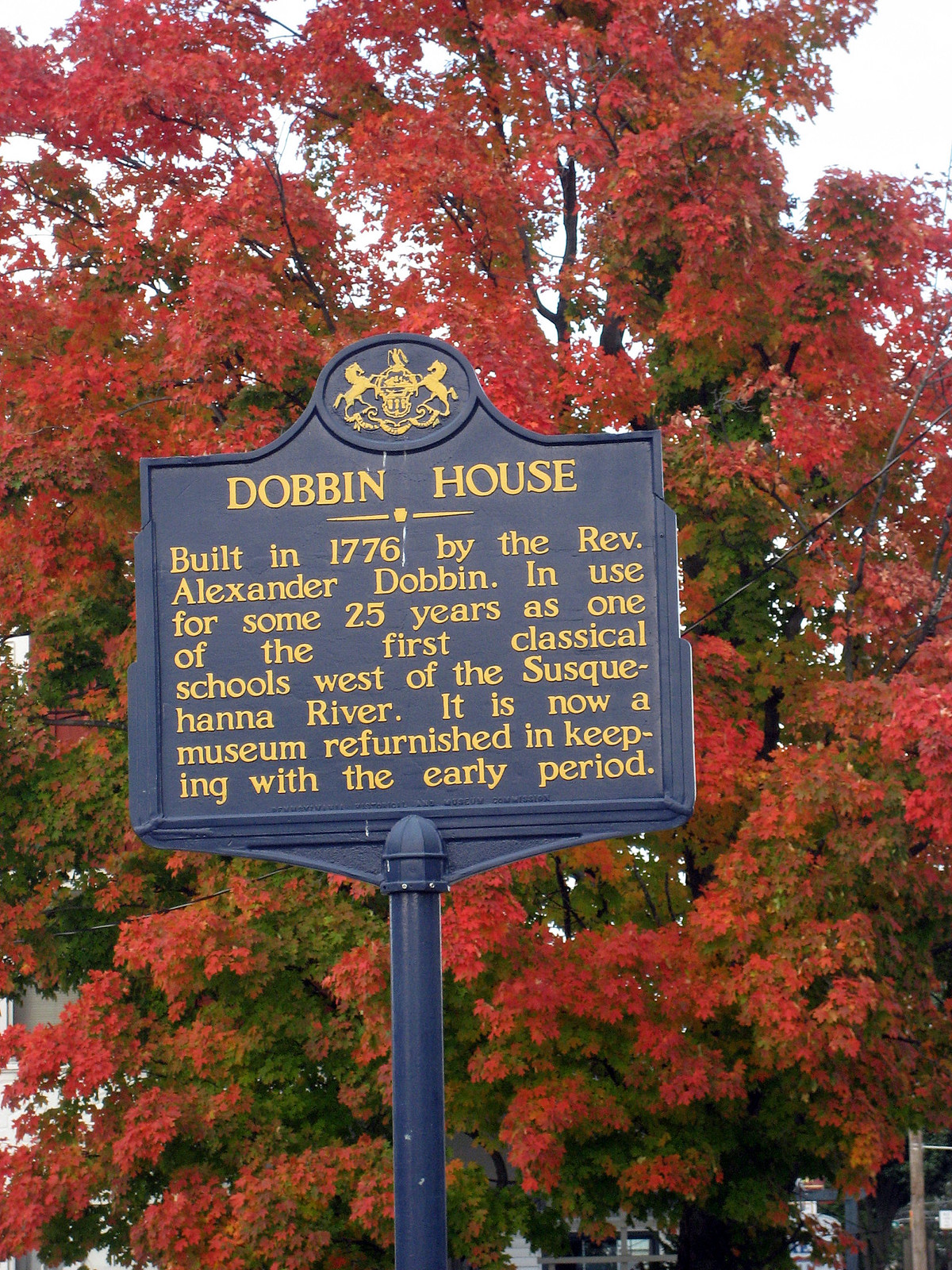In this vibrant scene, a towering maple tree, resplendent with a mesmerizing blend of bright red and green leaves, serves as a picturesque backdrop. In front of the tree stands a distinctive dark blue metal sign, adorned with elegant gold writing. At the top of the sign, there's an intricate circular emblem depicting two horses rearing on their hind legs, pressing against a central symbol. This historic marker provides details about the Dobbin House, proudly stating that it was built in 1776 by Reverend Alexander Dobbin. The house, which served as one of the earliest classical schools west of the Susquehanna River for around 25 years, has now been meticulously refurnished to reflect its original period and operates as a museum. The combination of the colorful foliage and the stately sign makes for a lovely and inviting scene, promising a fascinating tour of the distinguished historical house.